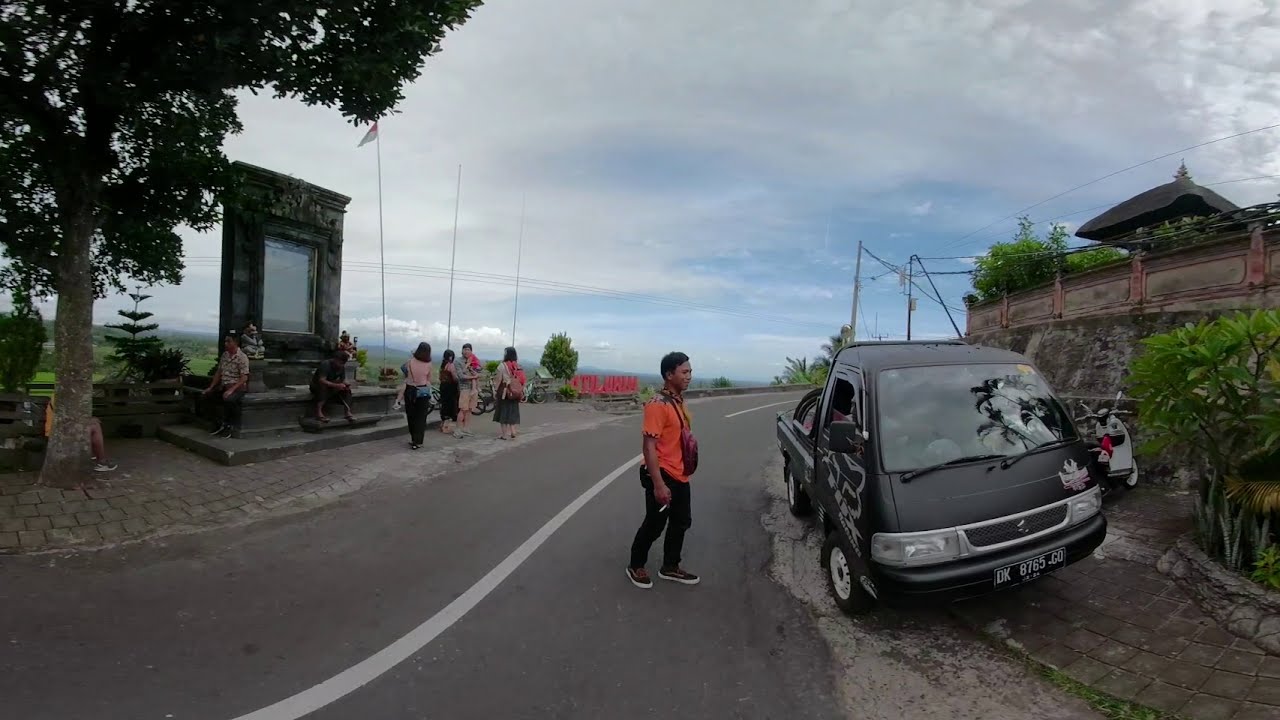The image shows a small two-lane road that winds from the left side of the picture, through the center, and off to the right. Standing in the middle of this road is a man with short hair, wearing black shoes, dark pants, and an orange short-sleeved shirt. He has a purple bag slung around his neck, which he holds down in front of him. Near him, towards the right side of the road, there's a small black truck with a truck bed, capable of fitting two people in the front. The truck has black wheels with white hubcaps and a license plate numbered DK 8765 GO. Next to the truck, there's a white and black two-wheeler vehicle. In the background to the right, there are some buildings including what appears to be a temple, along with trees and small shrubs. A small wall topped with a wooden railing and the roof of a hut can also be seen on this side. On the left side of the road, there are large cobblestones forming a sidewalk where people are standing. Adjacent to this sidewalk, there's a conspicuous monument or shrine with a few steps leading up to a large square feature, around which several people are gathered. Additionally, there's a large tree and a small unidentified structure with people nearby. The sky above is blue with some white clouds.